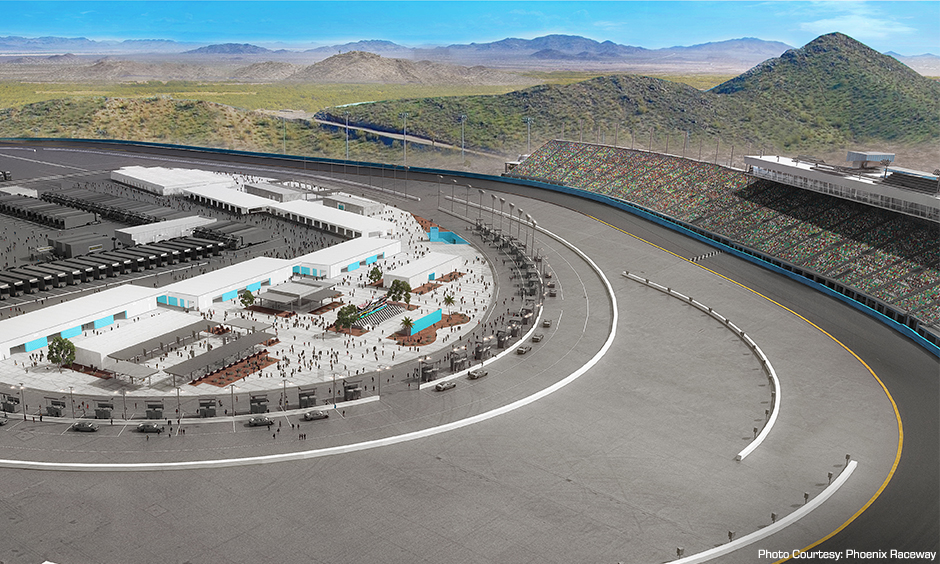This image presents a detailed, AI-generated racetrack set against a backdrop of green hills and mountains. In the foreground, on the right-hand side, there is a cluster of stadium seating, complete with areas at the top likely designated for race broadcasters. The track itself is oval-shaped, marked with white lines, and circles around a bustling pit area central to the scene. Here, numerous simulated people and cars are visible, interspersed among various buildings, some gray and white, and clusters of green trees. The pit area includes what appear to be fuel stations and is surrounded by a large number of tiny figures. The backdrop features both lush green mountains and darker, rocky peaks, with a slice of blue sky peeking over the horizon. A distinctive feature in the bottom right corner of the photo reads "Photo Choristy Phoenix Raceway." The overall image bears a surreal quality, blending realistic and artificial elements seamlessly, giving it an almost scale-model-like appearance despite its apparent vastness.